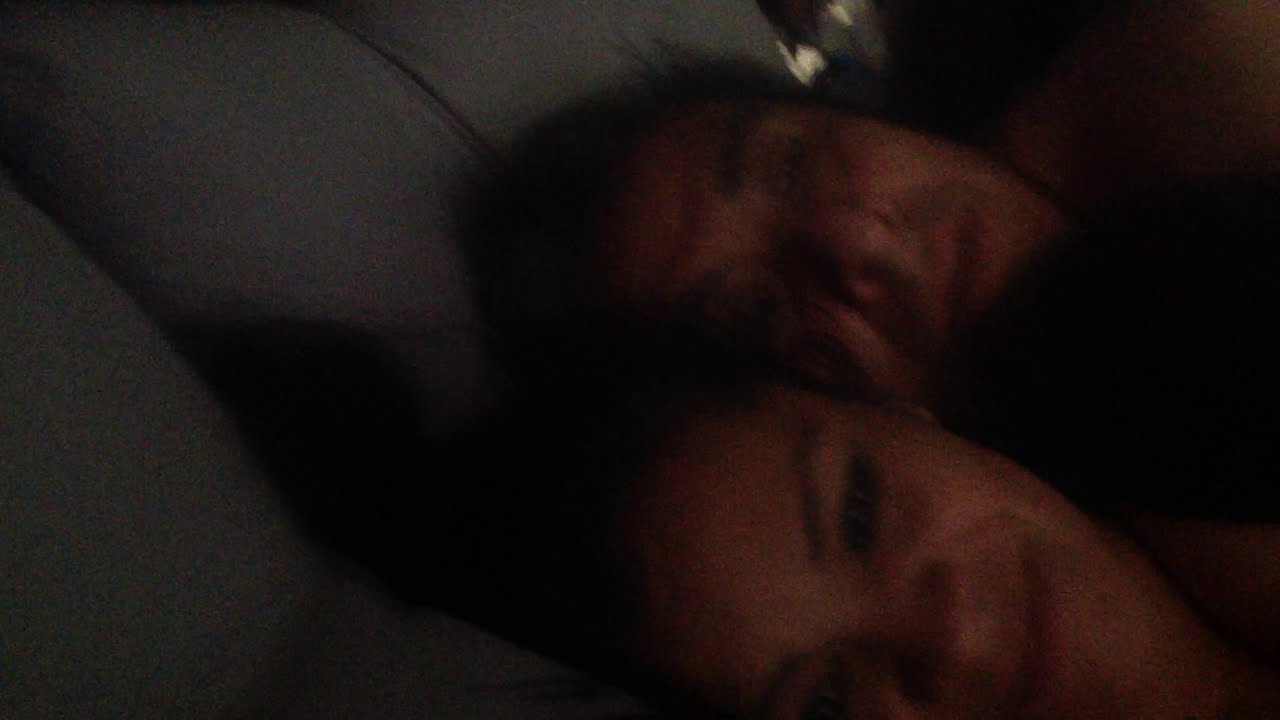In the dimly lit, indoor setting, a very blurry and indistinct photograph captures an intimate moment between two people resting close together. The woman, positioned in the bottom right of the image, has fairly brown skin, black hair, partially closed eyes, a black eyebrow, and a slight grin on her face. Behind her, the man with lighter brown skin, brown hair, and a mustache, rests his head, his eyes closed. Both figures are shadowed, making it difficult to discern the color of their shirts or additional details. Their heads lie on a gray pillow with subtle line patterns, filling the center left of the image. In the upper background, a light yellow blotch possibly represents an overhead light, casting minimal illumination on the subjects. The scene is enveloped in darkness with obscure surroundings, creating an intimate and cozy atmosphere as the two figures lay side by side, their bodies extending beyond the frame to the right.